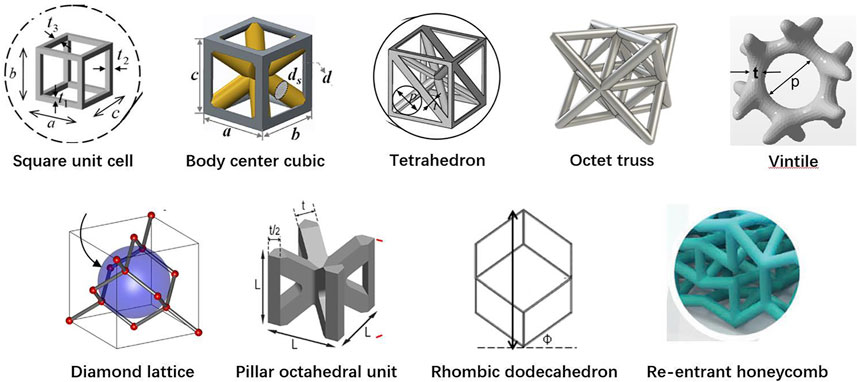This illustration features nine distinct three-dimensional geometric designs arranged in two rows, with five designs on the top row and four on the bottom. Each design is labeled with its respective name.

1. **Square Unit Cell**: A transparent 3D cube structure showcasing its outer edges.
2. **Body Centered Cubic**: Another cubic structure with internal spokes extending towards the cube corners.
3. **Tetrahedron**: A form featuring tetrahedral shapes with interconnected metallic sections.
4. **Octet Truss**: Resembling a rotated Rubik's cube, this design features angular supports.
5. **Ventile**: A complex structure with a circular spindle and irregular edges, akin to a teething toy.
6. **Diamond Lattice**: Displays a delicate wireframe cube with red nodes at connection points and a central purple sphere.
7. **Pillar Octahedral Unit**: Features a pentagonal structure with supportive pillars converging into its center.
8. **Rhombic Dodecahedron**: Illustrated as an upright open box, revealing its inner dimensions from a top-down perspective.
9. **Re-entrant Honeycomb**: A teal graphic design with interconnected geometric patterns.

The designs employ various shades of gray, yellow, teal, and purple, with some illustrations including dimension markings to indicate size and proportion. These graphics appear to be rendered using advanced 3D graphic software, suggesting scientific or material-based applications.